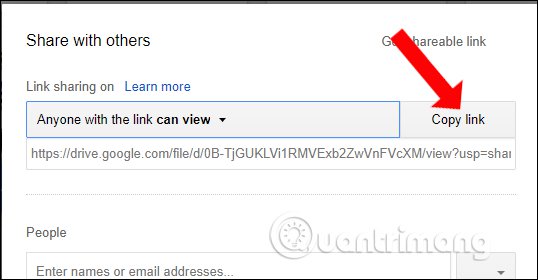The image displays a screenshot of a web page, framed with a black rectangular border. At the top of the page is a thin, black bar stretching the width of the screen. On the bottom right corner, there is a circular logo accompanied by the text "U A N T R I M A N G." The predominant background color of the webpage is white.

In the top-left corner, the words "Share with Others" are displayed prominently. At the top right, partially obscured text is followed by the words "Variable Link." A red arrow, pointing downward, directs attention to the phrase "Copy Link." Directly below "Share with Others," there is a link that begins with "Sharing on" and suggests to "Learn more." Following this, text indicates that "Anyone with the link can view."